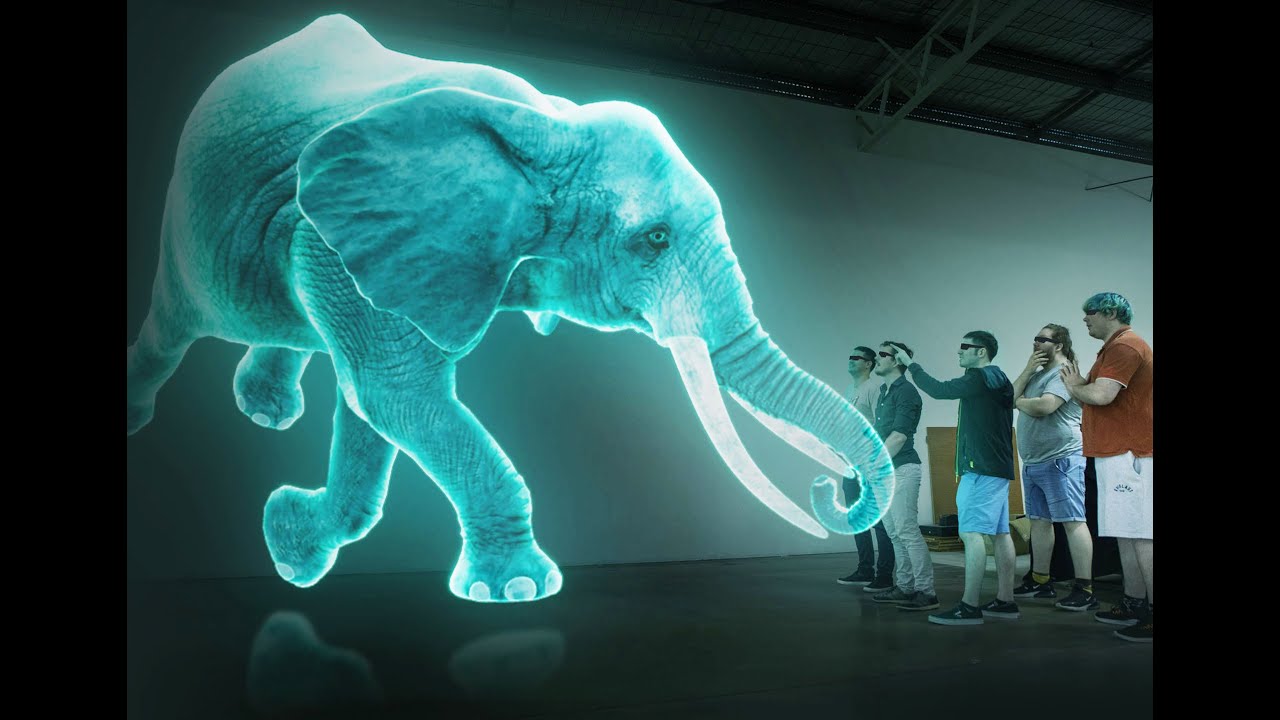The photograph captures a demonstration of augmented reality (AR) on a stage with a stark contrast between the white wall and the black floor. To the left, a large, semi-transparent, green-hued elephant hologram with visible tusks appears to float, its glowing presence creating an aura of luminescence. The elephant’s trunk extends towards five young men standing on the right, all seemingly captured in an interactive moment. Each man is equipped with identical black AR glasses, which contribute to the illusion of them witnessing the holographic elephant directly. Their reactions vary, with one man pointing and another appearing astonished with his hand on his jaw. The group is casually dressed, including attire such as red, gray, and black shirts, alongside a mix of shorts and pants. This detailed setup, along with the specific clothing and accessories, serves to profoundly illustrate the concept of AR, making the visual depiction both vivid and instructive.